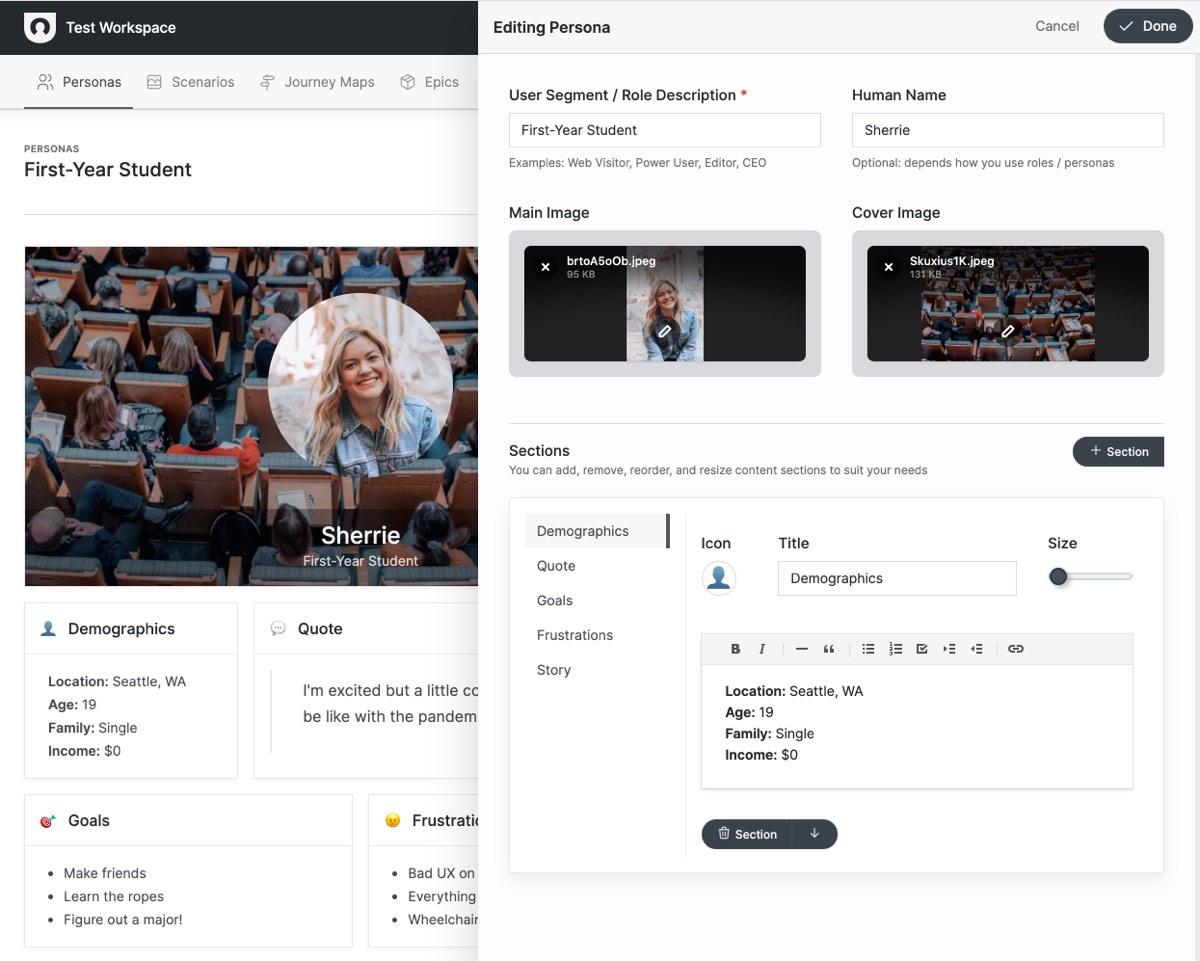This image comprises two overlapping screenshots related to a persona tool. The overlapping image on the right covers part of the one on the left. The left screenshot offers a structured view of various persona-related components within a workspace titled "Test Workspace." 

It includes categories such as "Personas," "Scenarios," "Journey Maps," and "Epics." Specifically featured is a persona named "First Year Student," represented by a profile centered in a circular photograph of Sherri, a young, blonde woman with long hair, who is smiling while wearing a denim shirt. The background captures an aerial view of numerous students seated with notebooks, tablets, and laptops.

The detailed persona description for Sherri includes:
- Name: Sherrie (S-H-E-R-R-I-E)
- Demographics: Location in Seattle, Washington, Age 19, Family status as Single, Income $0
- Goals: Make Friends, Learn the Ropes, Figure Out a Major

Both her quote and frustrations are partially obscured by the overlapping right screenshot.

The right screenshot, titled "Editing Persona," offers editing tools and options for the persona "First Year Student." It provides details specific to Sherrie's persona, such as:
- User Segment/Role Description: First Year Student
- Human Name: Sherrie (S-H-E-R-R-I-E)
- Customizable sections: Demographics, Quote, Goals, Frustrations, Story

Highlighted elements include "Demographics" selected with title, location (Seattle, Washington), age (19), family status (Single), and income ($0). It notes that users can add, remove, reorder, and resize content sections to tailor the persona as needed.